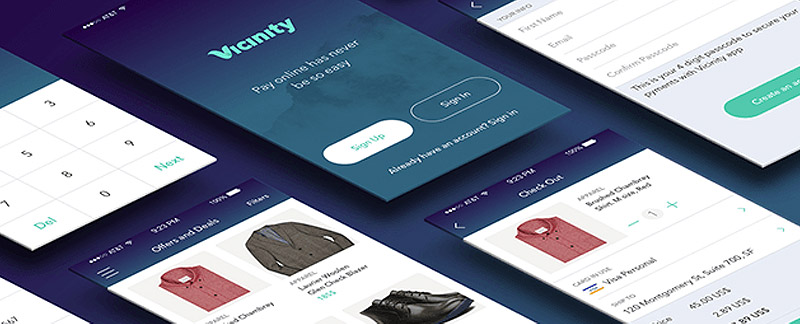This advertisement for Vicinity showcases various screenshots from a mobile phone, highlighting the ease of their "Pay Online" service. The central screenshot prominently displays the slogan "Pay online has never been so easy" and options for "Sign Up" and "Sign In" for users to access their accounts. The service provider AT&T, time of 9:23 p.m., and a fully charged battery are also visible, suggesting a seamless user experience at any time.

Several other screenshots illustrate additional functionality: one shows a virtual shopping cart with a user browsing through clothing items such as a maroon shirt, a gray shirt, and black shoes, under the header "Offers and Deals." Another screen shows fields for setting up login information, including first name, email, and password. Additionally, there's a snippet of a virtual keypad with the characters 7580 and 369 visible, hinting at in-app calculations or number entry. Together, these screenshots effectively depict Vicinity's user-friendly platform that integrates online shopping and secure payment options, emphasizing its comprehensive, mobile-centric design.